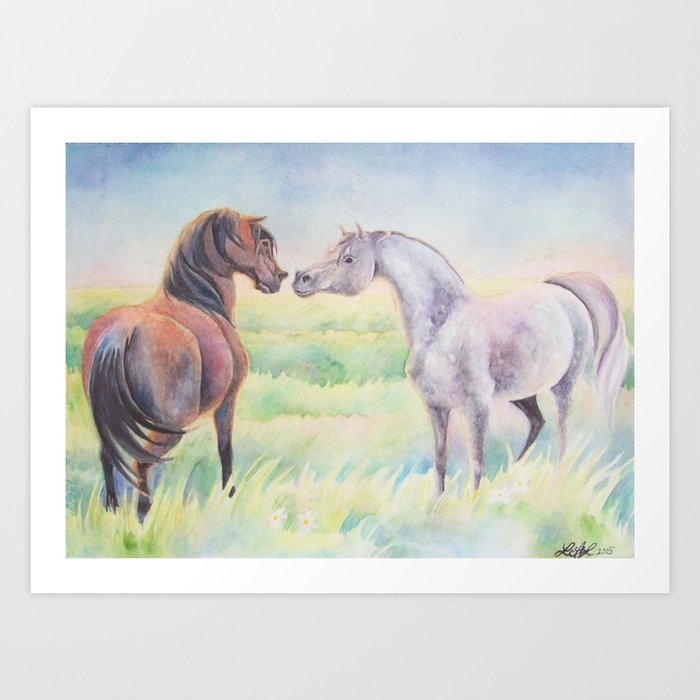This is a detailed watercolor painting, possibly done with colored pencils, mounted on a light grey wall in a sheer white frame with a one-inch border. The rectangular image depicts two horses situated in a field of light green and bluish grass, interspersed with small white flowers. The sky above is a blend of whitish, bluish, and grayish hues, adding a somewhat cloudy atmosphere.

On the right side of the painting is a near-white horse with subtle pink accenting and a white mane and tail. This horse is facing leftward, its expressive eyes looking slightly downward. Meanwhile, the brown horse with a black mane and tail is positioned with its rear towards the viewer and its head turned back towards the white horse, seemingly about to meet its gaze. This brown horse, described as having a walnut-like hue, has its tail flicked in motion and its posture indicates a dynamic interaction with its counterpart. Notably, the white horse has its left back leg raised, contributing to the scene's sense of movement and connection between the two animals.

The piece also features a prominent signature in the bottom right corner, which appears to start with an "L" and is dated 2015. The overall artistic style leans towards the cartoonish, with an almost whimsical portrayal of the natural elements and the figures of the horses.